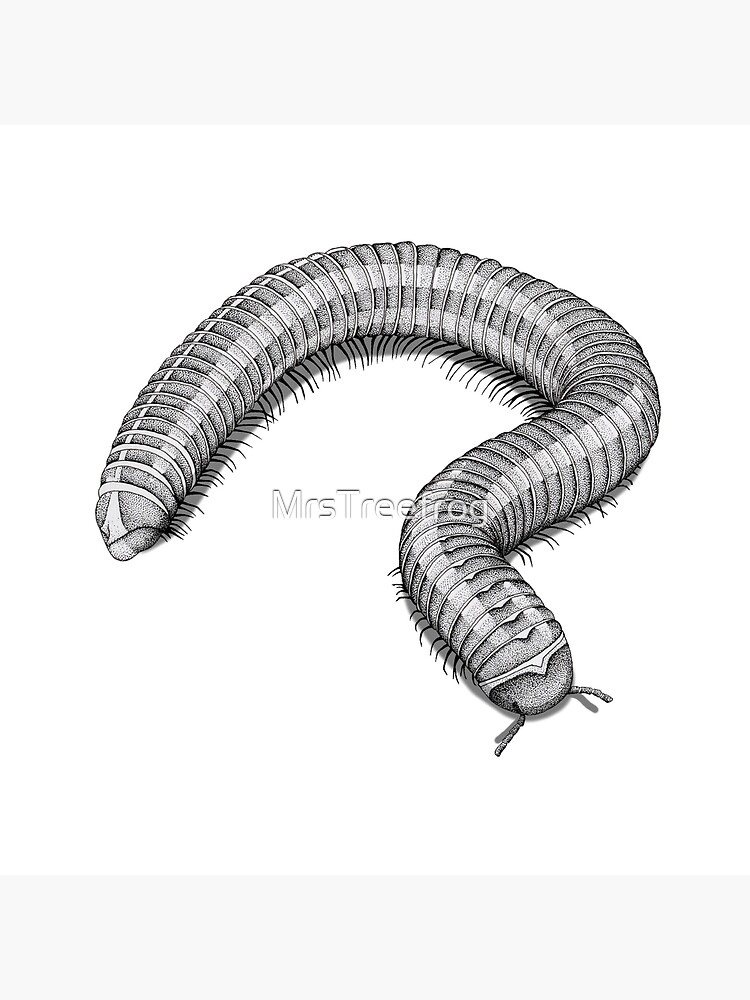This image is a detailed pen and ink drawing of a millipede, noticeably rectangular and taller than it is wide. The illustration is set against a plain off-white background with slightly darker top and bottom borders. The millipede features intricate detailing, showcasing numerous pairs of tiny black legs, segmented body parts, and two pairs of antennae. Its body exhibits fine dot shading for depth and texture, with white stripes running longitudinally along its sides. A thin, delicate line starts from its tail and extends partially along its body. The millipede's head, marked by small eyes and whisker-like antennae, is positioned in a question mark shape. Prominently across the center of the image, including partially over the millipede, is a watermark that reads "Mrs. Treefrog" in see-through black letters.